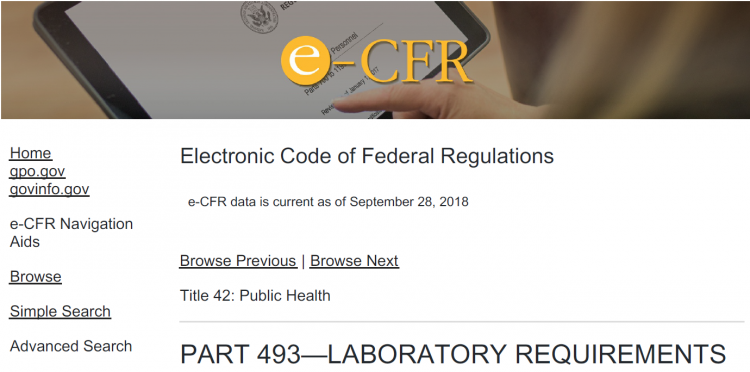The image appears to be a screenshot from a web page or a PDF document, featuring the Electronic Code of Federal Regulations (e-CFR). At the top of the image, there is a logo consisting of a small letter "e" inside a yellow circle, followed by a hyphen, and the capital letters "CFR". Behind this logo, a person's hand is seen interacting with a tablet, which displays an official-looking document marked with a seal.

Below the logo, the text reads: "Electronic Code of Federal Regulations." It further specifies that the e-CFR data is current as of September 28, 2018. In the center of the image, there are hyperlinks labeled "Browse Previous" and "Browse Next". The current section displayed is "Title 42: Public Health", specifically focused on "Part 493: Laboratory Requirements".

On the left-hand side of the image, there is a vertical menu with several navigation links, including "Home", "gpo.gov", and "govinfo.gov". Beneath these links, there is a section titled "E-CFR Navigation Aids" with additional links for "Browse", "Simple Search", and possibly "Advanced Search", although the advanced search link is not visibly underlined to confirm its hyperlink status. The screenshot is cut off, obscuring any further details.